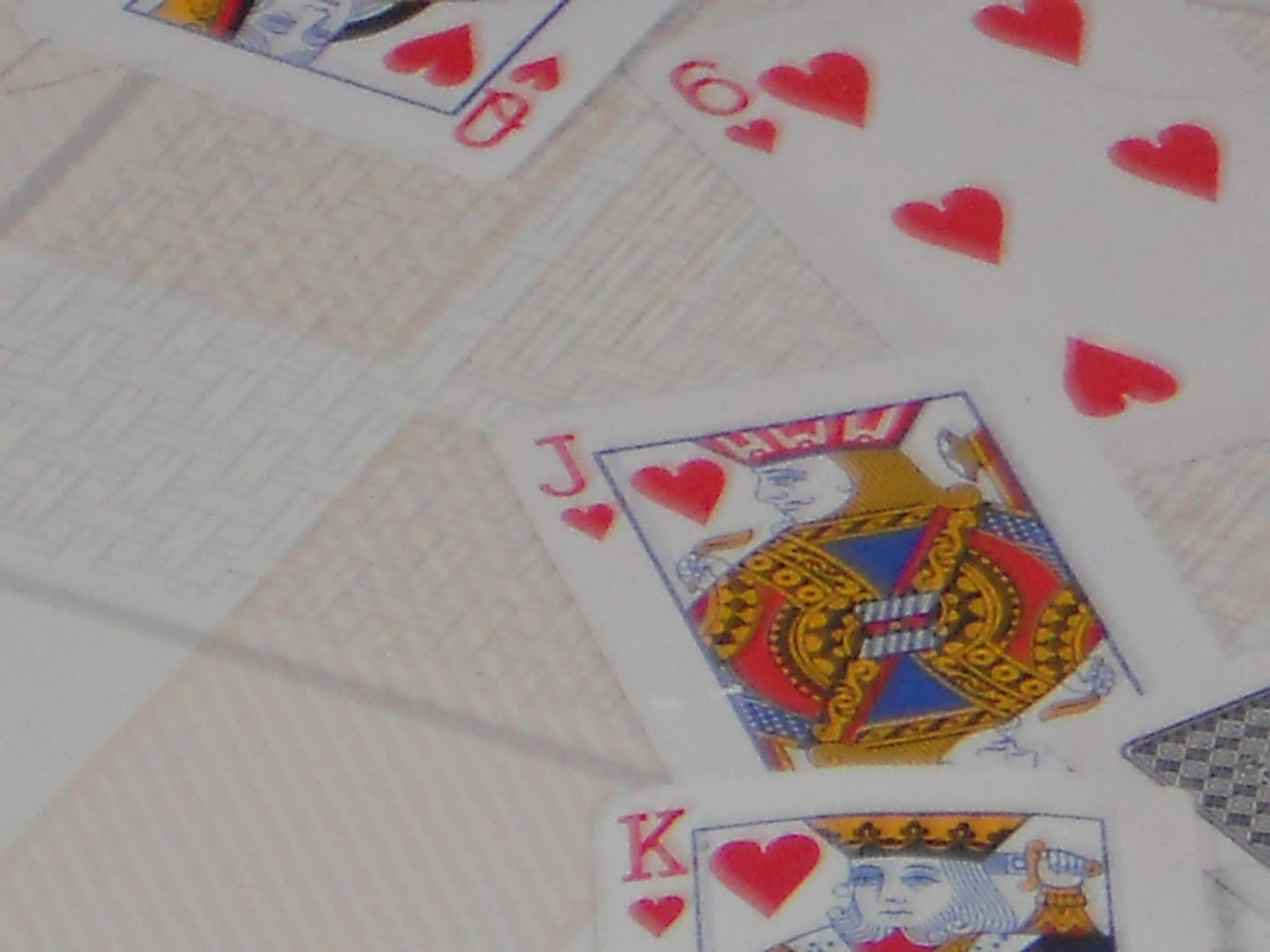A slightly fuzzy image showcasing an assortment of playing cards arranged on a checkered backdrop. At the top of the picture, the partial visage of the red Queen of Hearts is visible, with just the upper portion of the Queen's head in view. Just to the right, the full face of the red Six of Hearts stands out more prominently. Below, the red Joker card is mostly visible, making its playful design discernible. Beneath the Joker lies a card flipped upside down, its black patterned back exposed. Further down, the top of the King of Hearts’ head can be seen, though the rest of his card is cut off by the edge of the image. The cards rest atop a checkered surface that alternates between shades of white and beige, with a subtle woven texture adding depth to the scene.